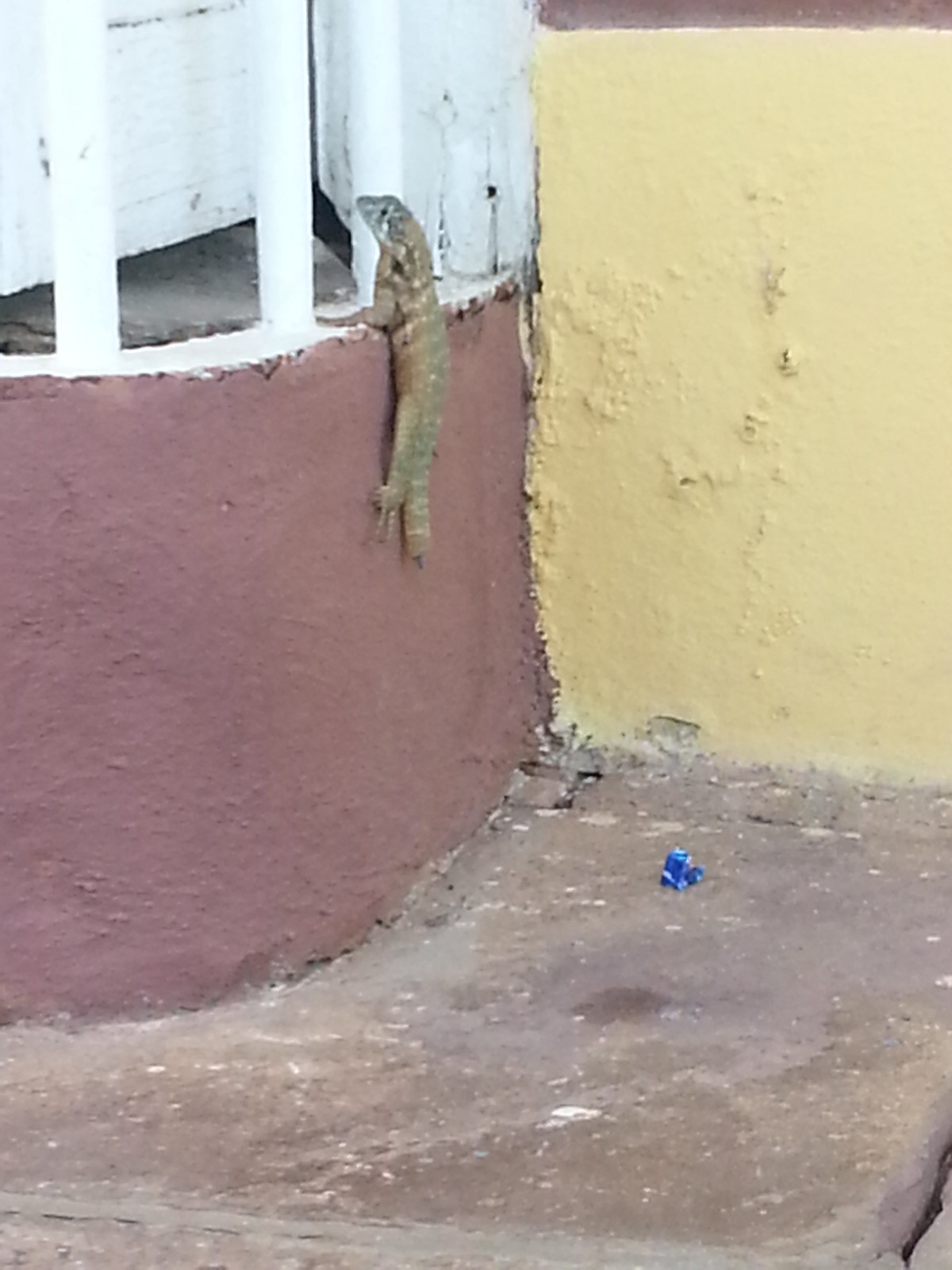In this detailed outdoor image, taken in the middle of the day, a dark tan lizard, possibly a gecko, with greenish-brown rings on its back and a partially regenerated tail, is prominently featured. The lizard, which has black eyes and a white-colored muzzle, is climbing up a wall made of stone painted in various shades of brown, yellow, gray, maroon, blue, and tan. It is positioned near the top left of the image, heading towards a balcony with white railings. The setting appears to be just outside a house or building, with the lizard’s front legs gripping the white rails above a chocolate brown concrete step. The scene, devoid of any text, captures the natural elements and structure of the building, emphasizing the stone materials and painted surfaces within the frame.